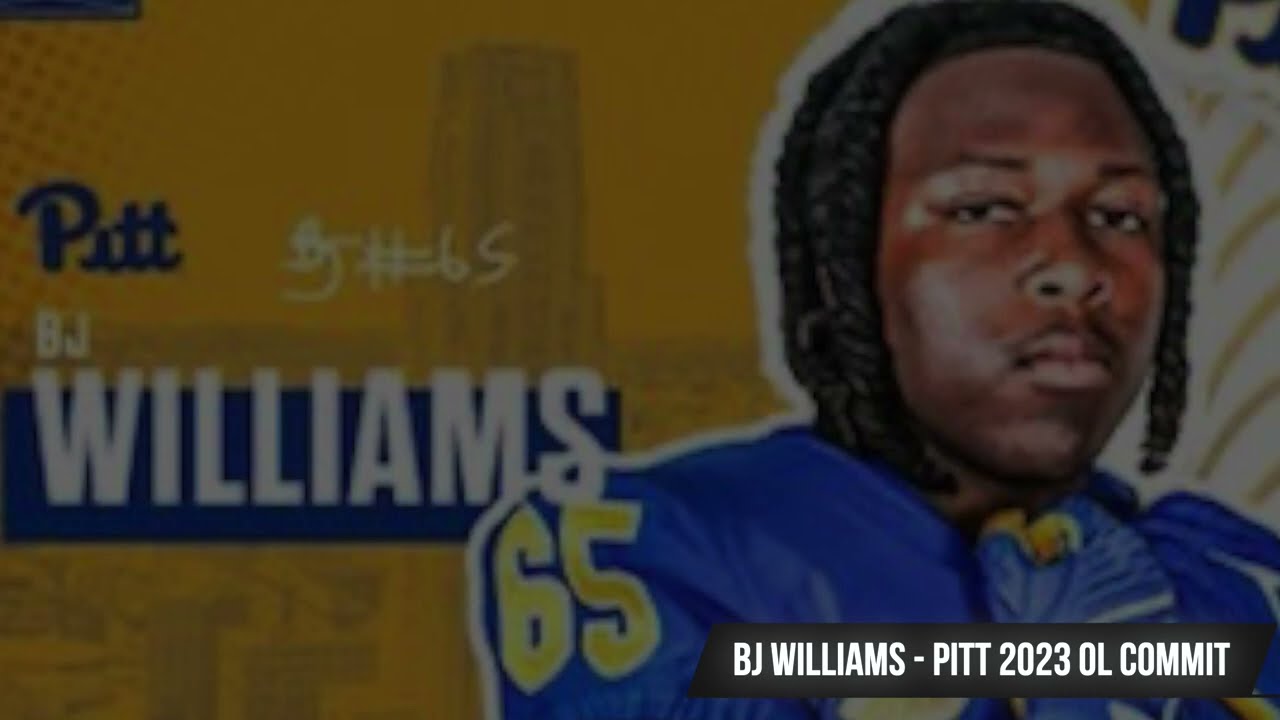The image shows an infographic featuring BJ Williams, a football player committed to the University of Pittsburgh for 2023 as an Offensive Lineman (OL). The background is a stylized yellow depiction of the city, highlighting the word "PITT" in bold blue letters. On the right side of the image, BJ Williams, an African American male, is prominently displayed. He has shoulder-length black braids and is wearing a blue jersey with the number 65 in yellow. Below the logo "PITT," his name “BJ Williams” is written in white with a blue stripe underneath. BJ Williams appears serious in his pose, and he also sports matching blue gloves. The text on the image clearly states: "BJ Williams Pitt 2023 OL Commit."